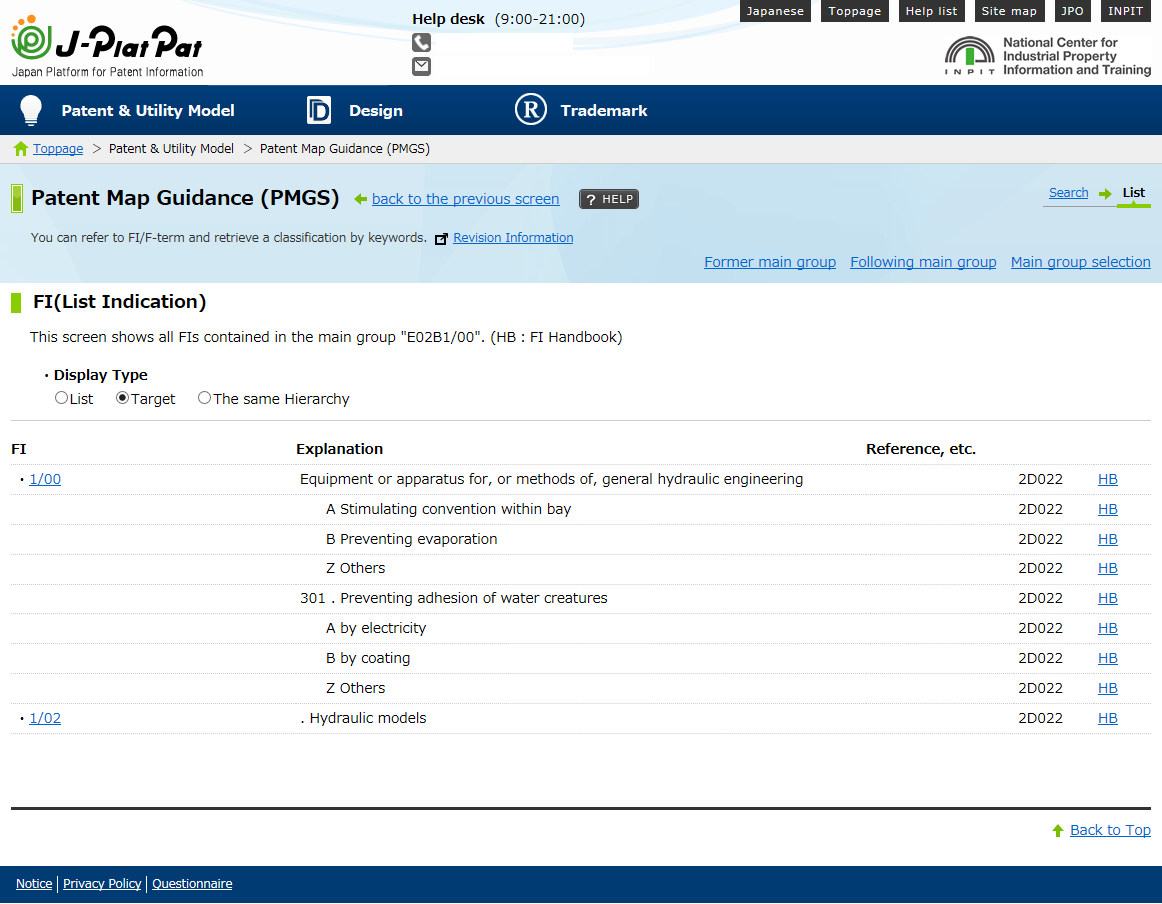The image showcases a webpage from the Japan Platform for Patent Information, detailing various functionalities and services available to users. The header highlights the helpdesk hours, which operate from 9 AM to 9 PM. The navigation includes options such as a help list, sitemap, and information about GPO and INPIT (National Center for Industrial Property Information and Training).

The webpage focuses on patent information, covering Patent and Utility Model, Design, Trademark, Patent Map Guidance, and more. There is a section that allows users to return to a previous screen and provides a reference for FI (File Index) classification retrieval using keywords.

Specific revision information is provided, along with details on the former and following main groups. The main group selection screen displays all FIs within the main group, exemplified by an FI code "E02BI / 00", categorized under "Display Type: List".

An explanation section describes the main group as concerning "Equipment or apparatus for or method of general hydraulic engineering," with subcategories such as "A: Stimulating convention within bay" and "Z: Others".

This organizational layout is designed to facilitate easy navigation and efficient retrieval of patent information, making it user-friendly for professionals engaged in industrial property and patent research.